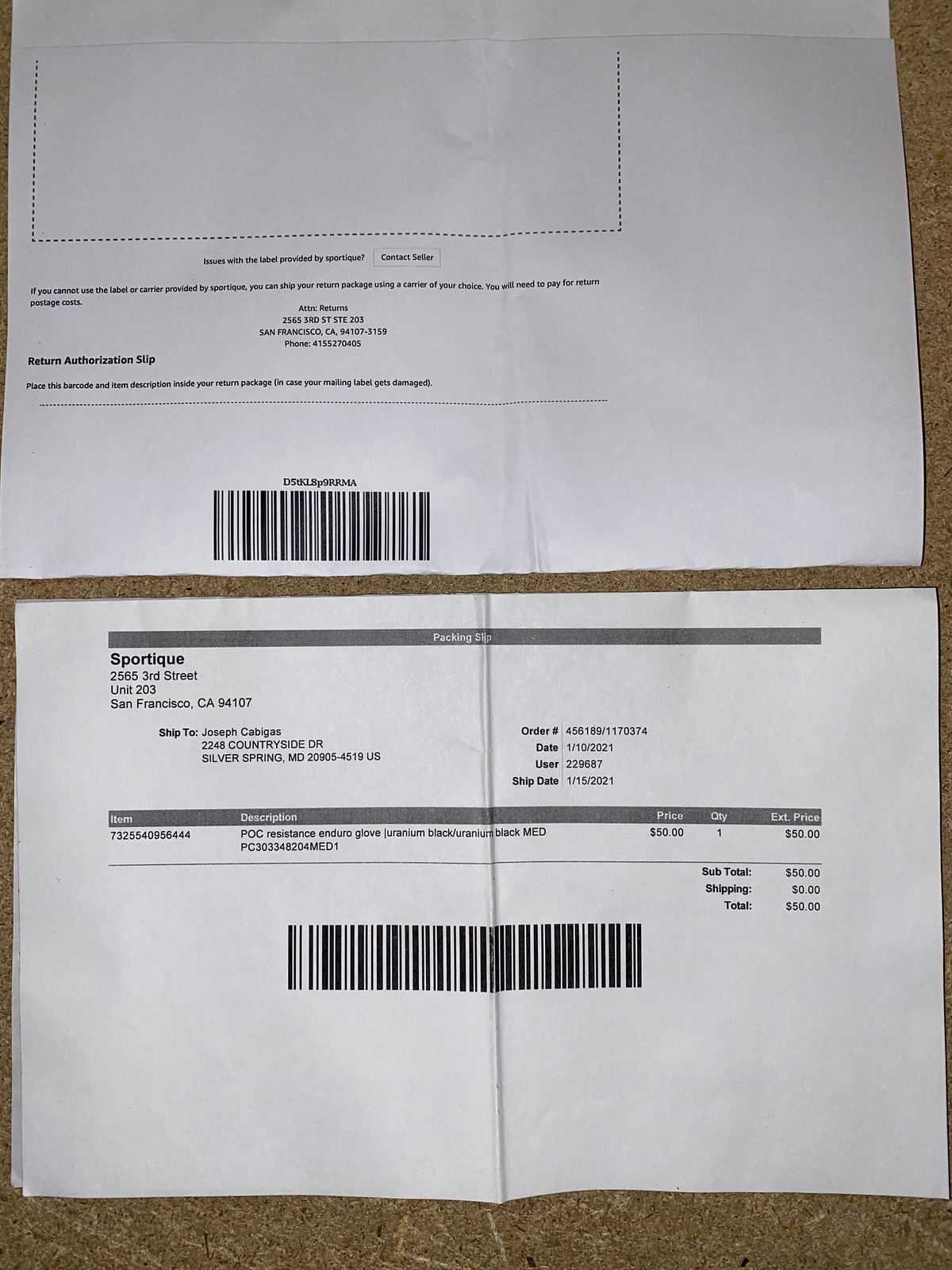This is a color photograph featuring two white labels on a brown, potentially wooden, background. The labels are positioned vertically, one above the other, with a noticeable gap revealing the brown background in the middle. The top label has a blank rectangle at the top and appears to have some faint, indistinguishable writing underneath it. Towards the center-left bottom edge of this label, there is a barcode. The bottom label features a prominent black bar at the top, beneath which appears to be an address. Additional text is visible towards the center and right of the label, accompanied by another black bar. This label likely serves as a receipt, with unreadable text and a total amount listed towards the right. A barcode runs through the middle section, and there is a noticeable fold line across the center of this paper, indicating it has been folded before.